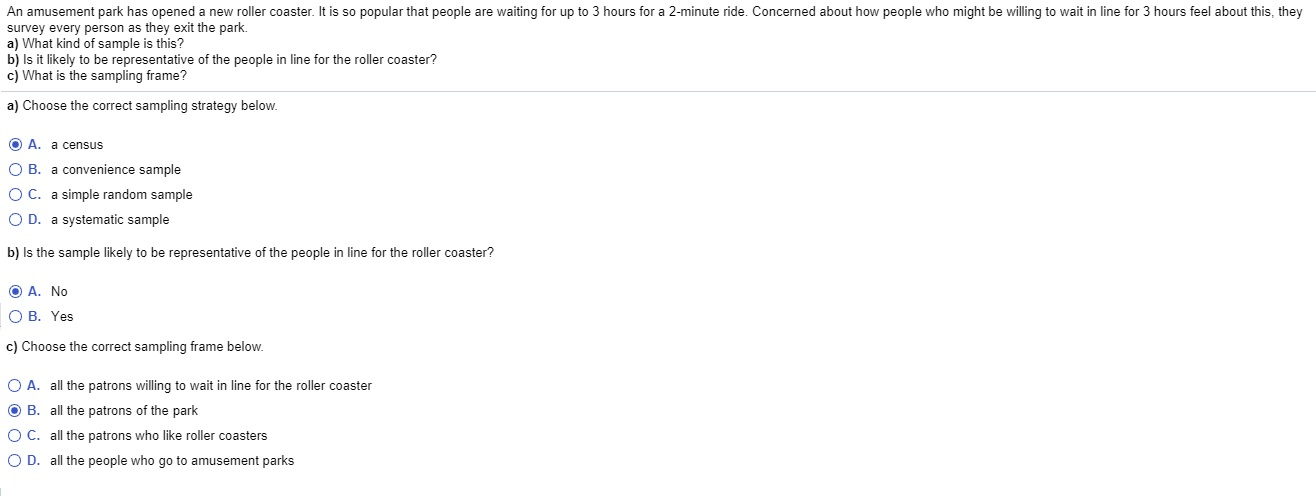A detailed caption for the provided image could be:

"A screenshot of an online test featuring a scenario about a new rollercoaster at an amusement park. The first question describes a scenario where the rollercoaster is so popular that people are waiting up to three hours for a two-minute ride. The park conducts a survey of every person as they exit the park to understand their feelings about the wait. The test then poses three sub-questions: 

A. What kind of sample is this? 
B. Is it likely to be representative of the people in line for the rollercoaster? 
C. What is the sampling frame?

The test taker selected "a census" for question A, "no" for question B, and "all the patrons of the park" for question C. Additional instructions ask to choose the correct sampling strategy and assess whether the sample is likely representative of those in line for the rollercoaster, as well as to select the proper sampling frame, all of which are tied to the initial options provided."